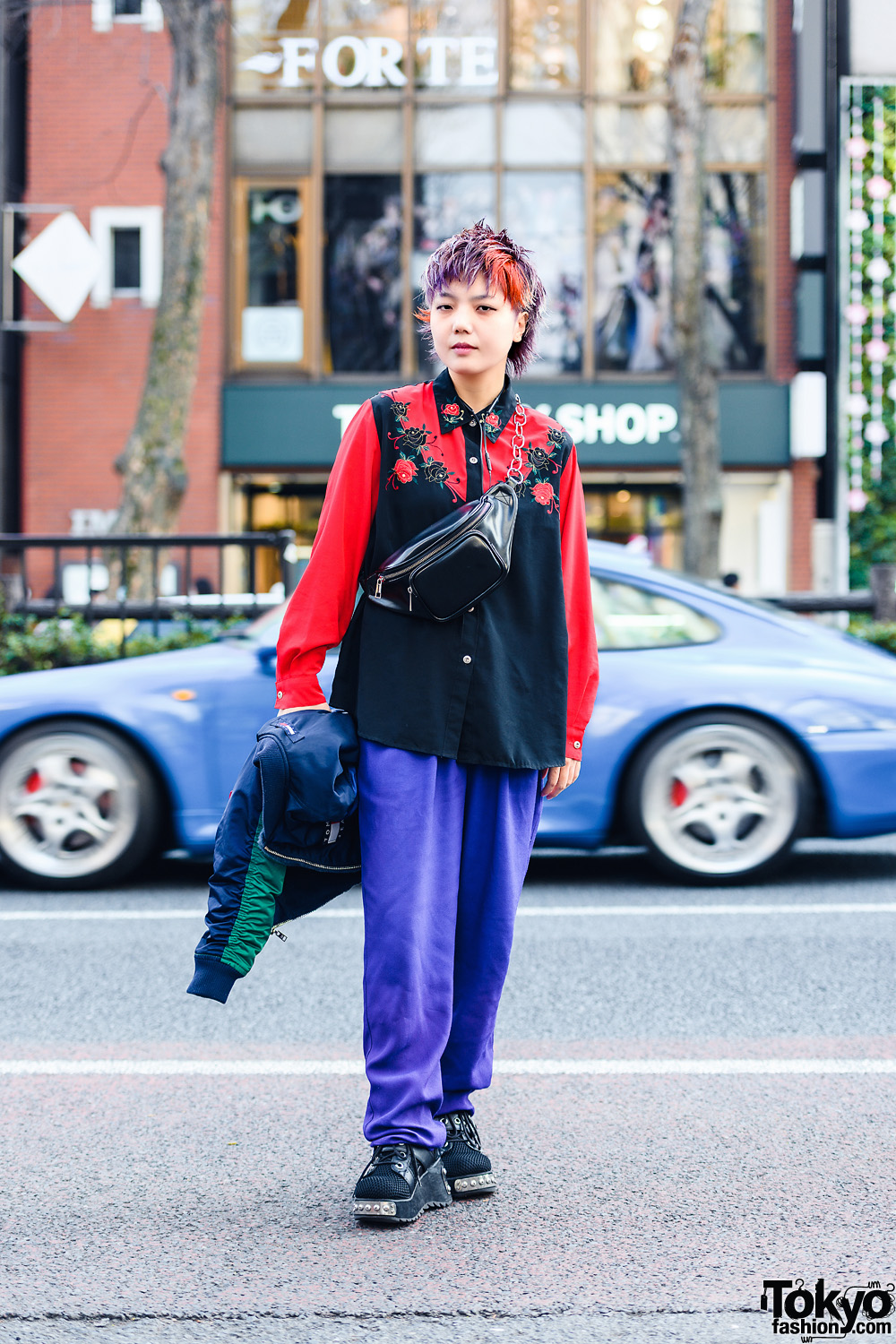A vibrant photograph taken during the daytime features a stylish young Japanese woman standing on a sidewalk in front of a distinctly colored light purple Porsche 911. The image, marked with the tokyofashion.com logo in the bottom right corner, showcases the woman’s striking fashion sense. She is wearing bright purple long pants and oversized black tennis shoes with large platforms. Her top is a long-sleeved black shirt adorned with red sleeves and a pattern of red roses on the chest. She accessorizes with a black fanny pack draped over her shoulder and neck. Her short, spiky hair is dyed a striking combination of purple and reddish hues. In her right hand, she holds a blue and teal biker jacket while her left hand rests casually by her side. The backdrop includes a tall red brick building with numerous windows, illuminated by sunlight, adding to the vibrant atmosphere of the scene.